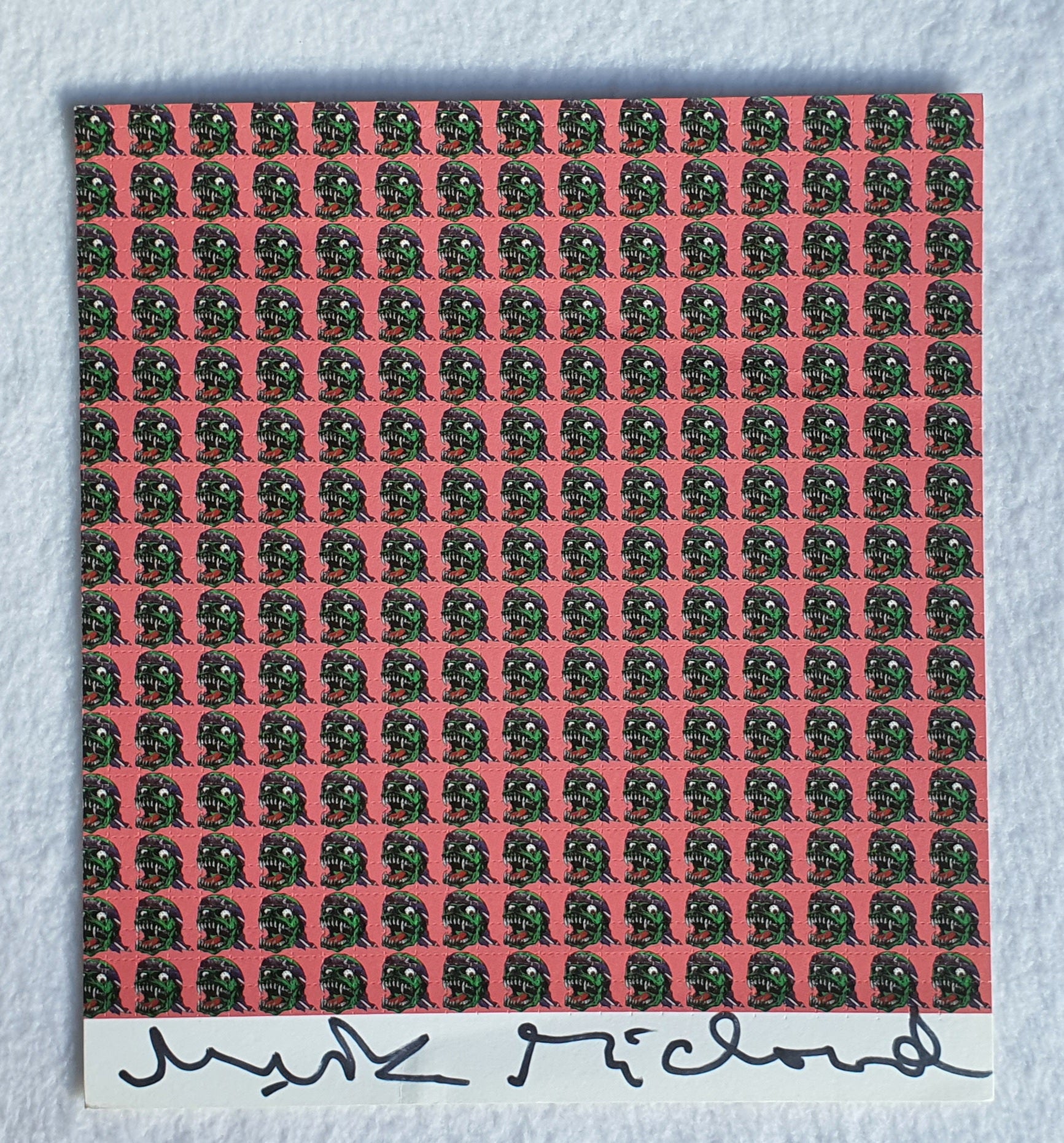The image resembles a striking record cover laid out on a white fabric background. It features a repeating pattern of 20-by-20 squares, each showcasing a green-faced zombie with sharp teeth, bulging white eyes, and a pink tongue sticking out of its wide-open mouth. The zombie head is adorned either with black hair or a helmet, and a bone—potentially a shoulder or neck bone—protrudes from the bottom. The background behind these zombie heads is predominantly pink. At the bottom of the image is an undecipherable signature in black ink; it's difficult to determine, but it appears to be a first name followed by "McCloud." The entire image is divided into numerous perforated squares, contributing to its unique texture. In the background, there is a white textured wall or fabric adding subtle contrast to the vibrant and macabre design.